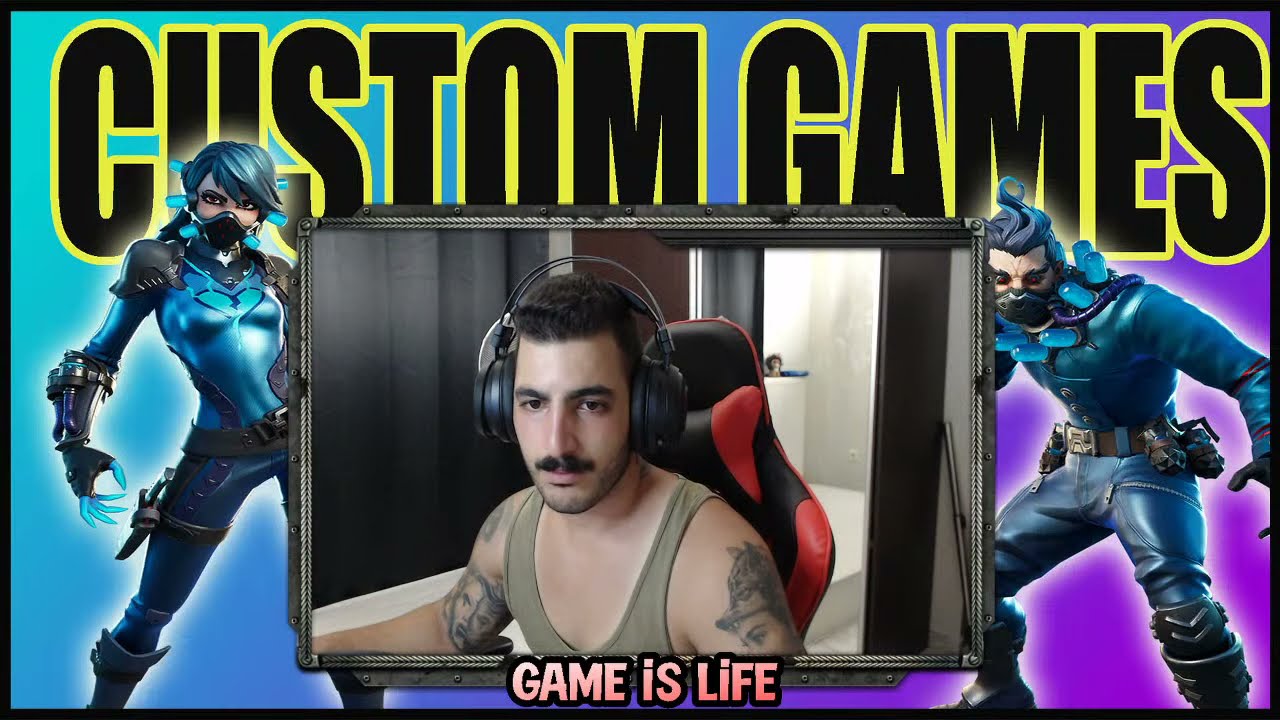This appears to be a screen grab from a live stream or a video thumbnail typically found on YouTube. At the top of the image, bold black and yellow text reads "Custom Games." Flanking the central frame, which features the streamer, are two video game characters. To the left, a female character sports blue hair, a black mask, blue and black armor with distinctive parts on her shoulders and thighs, and spiky fingers. On the right, a male character dressed similarly in blue and black armor, with knee guards and what seem to be grenades attached to his belt, also wears a mask and has hair styled in a man bun or spiked upwards.

The central figure is a young man, likely in his mid-20s, sitting in a black and red gaming chair. He wears a gray-green tank top that reveals tattoos on both arms, has short dark hair, a mustache, and light facial hair. He is wearing headphones, suggesting he is actively engaging in the game. The streamer’s image is enclosed within a border that gives off a techy vibe. Beneath this central frame, a caption reads “Game is Life.”